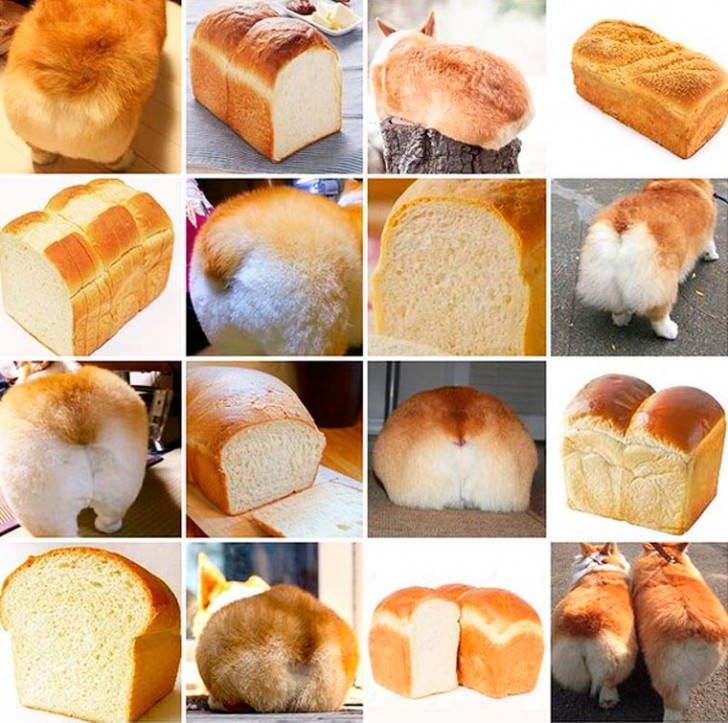The image is a grid consisting of 16 squares, arranged in four rows and four columns, creating a checkerboard pattern. Each square alternates between an image of a brown dog’s rear end and various forms of white bread, with careful attention to detail contributing to the surprisingly similar appearances in shape and color. The sequence starts from the top left with a brown dog's rear end, followed by a loaf of white bread, then a dog on a log, and another loaf of bread. The second row presents a loaf of sliced white bread, a brown and white dog's rear end, another loaf of sliced white bread, and a different dog’s rear end. The third row also alternates with a dog’s rear end, a loaf of sliced bread, another dog’s rear end, and another loaf of bread. The final row continues the alternation beginning with bread, then a dog’s rear end, another bread loaf, and ends uniquely with two dogs. The consistent pattern highlights the similarity in color and form between the dogs' rear ends and the loaves of bread, creating an amusing and visually intriguing montage.